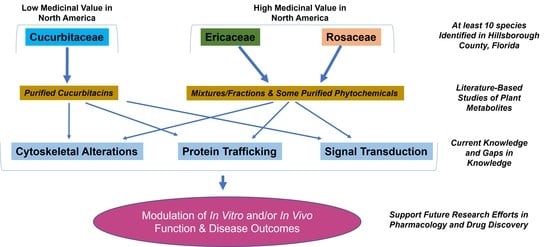The image depicts a detailed flowchart on a white background, illustrating the modulation of in vitro and in vivo function and disease outcomes, structured around multicolored rectangles connected by arrows. At the top left, there’s a blue box labeled "Curcubitaceae," with an arrow leading down to a yellow box labeled "Purified Cucurbitacins," and further down to a light blue box labeled "Cytoskeletal Alterations." On the top right, a green rectangle labeled "Ericaceae" points to a yellow rectangle labeled "Mixtures Fractions and Some Purified Phytochemicals," which then branches out with two arrows leading to light blue boxes titled "Protein Trafficking" and "Signal Transduction." Adjacent to the green rectangle is a pink rectangle labeled "Rosaceae," also pointing down to the same yellow rectangle. Centrally positioned, the chart emphasizes a comparison of medicinal value in North America, with high medicinal value noted in certain boxes. At the bottom, a prominent pink oval outlines key concepts: "Modulation of In-Vitro and In-Vivo Function and Disease Outcomes." On the right side, smaller black text highlights supporting statements: "At least 10 species identified in Hillsborough County, Florida," "Literature-Based Studies of Plant Metabolites," "Current Knowledge," and "Gaps in Knowledge," collectively endorsing "Support for Future Research Efforts in Pharmacology and Drug Discovery."